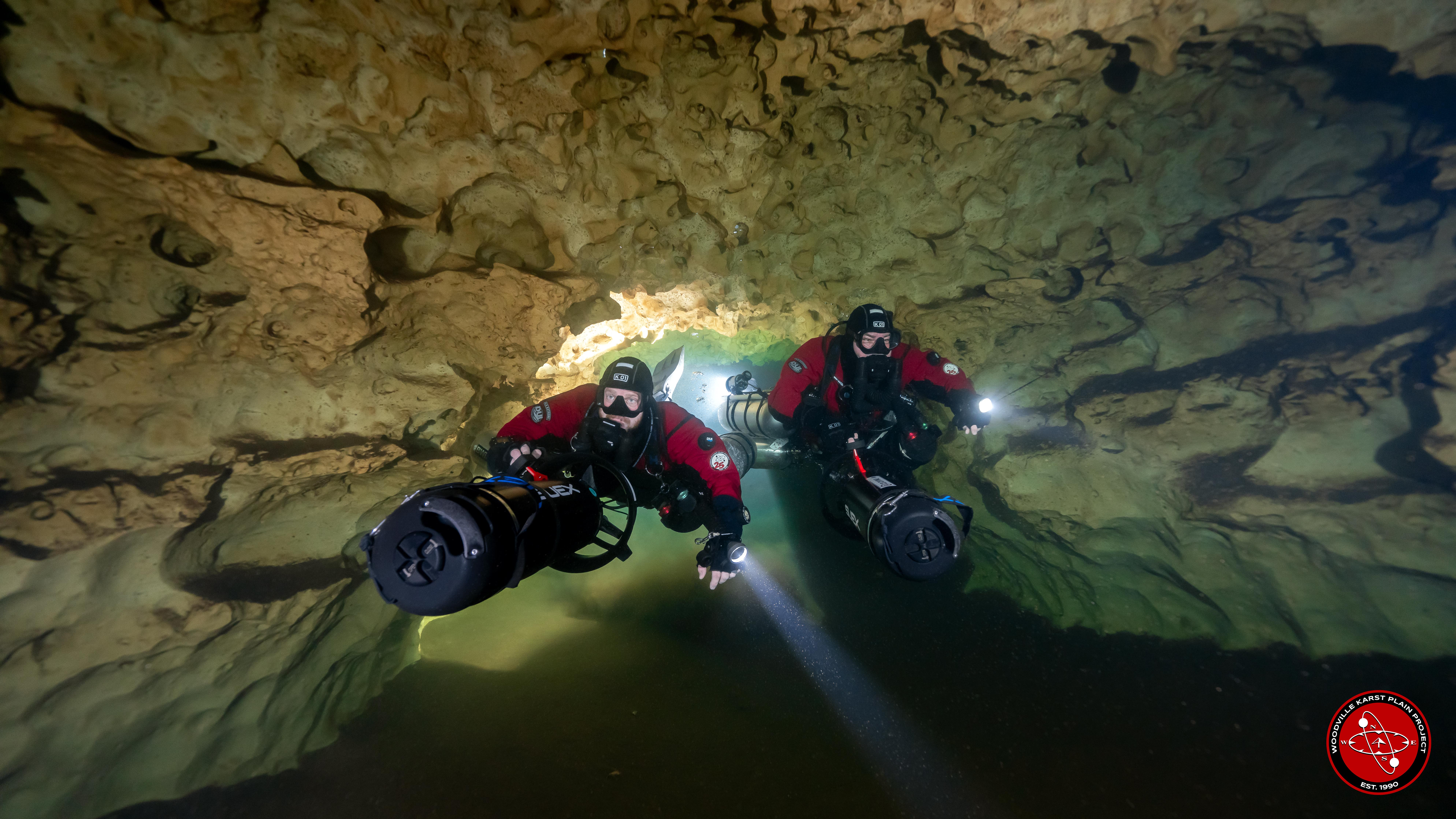The image depicts two underwater cave divers fully equipped with scuba gear and various lights illuminating their path. Their red, heavy-duty diving suits contrast with the black helmets and partial gloves they wear. Both divers are holding cylindrical underwater propulsion units, labeled "U-E-X," which assist their movement through the clear, freshwater of the limestone cave. The cave’s walls feature shades of tan, brown, and hints of green, suggesting an environment similar to the springs found in Florida. Each diver has flashlights affixed to their left wrists, casting beams through the serene, fishless water. One diver appears to be dragging a pack behind him. In the lower right corner of the image, there is a logo for the Woodville Karst Plain Project, established in 1990, which includes a gimbal with a navigation compass and orbiting particles.